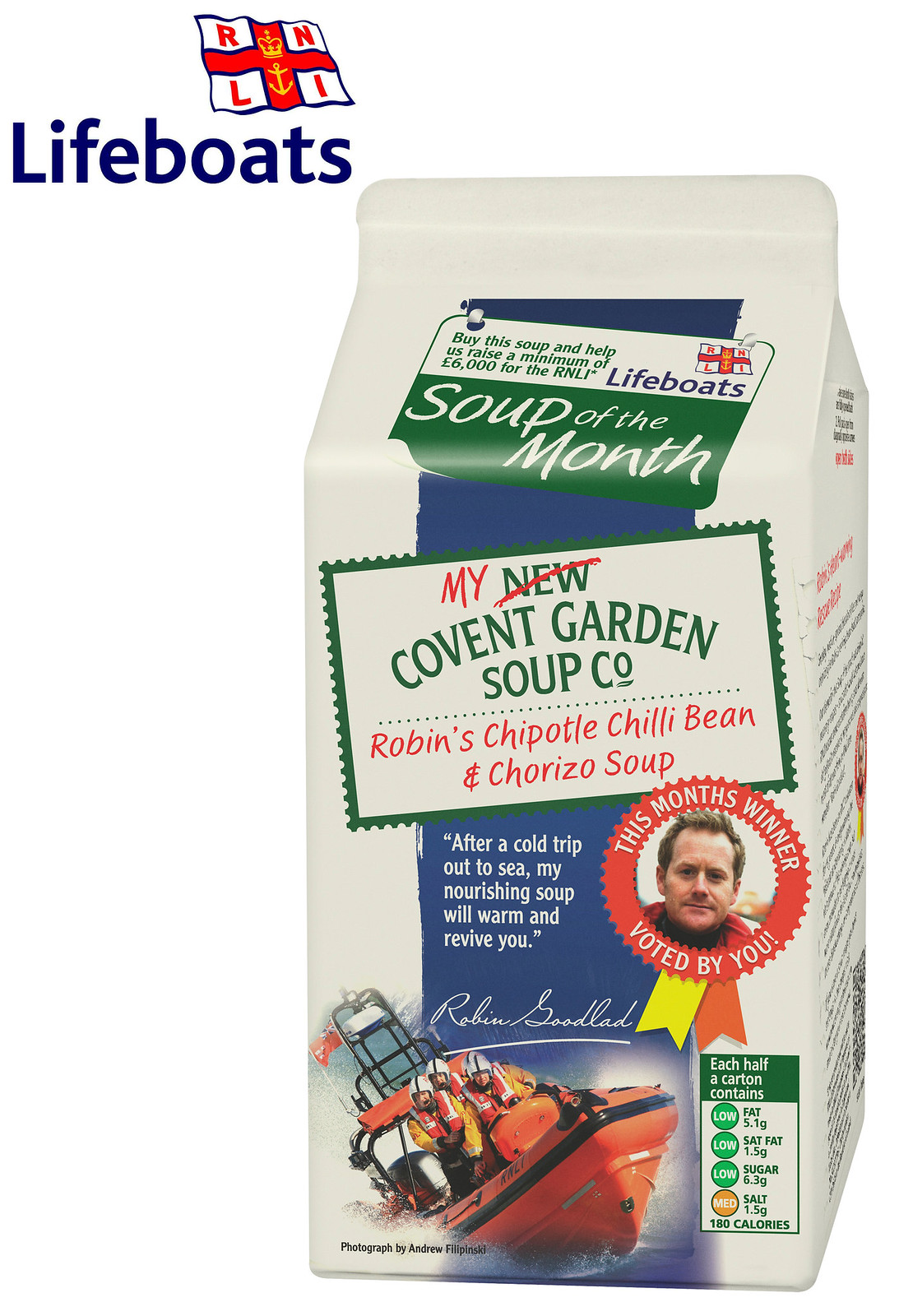This image displays a detailed design of a white soup carton, styled like a traditional milk carton, under the theme "Lifeboats". At the top left, a waving flag decal features an anchor and crown in its center. Below, blue text titles this product "Lifeboat Soup of the Month". A notable image of a headshot of a white man with brown hair, dressed in red clothing, is enclosed in a red circle. Surrounding this photo, the text states "This Month's Winner Voted By You" with his signature, Robin Goodland, underneath.

Covering the carton, numerous vibrant colors and framed information pieces create a lively, informative design. Centralized text reads "My New Covent Garden Soup Co." with 'New' crossed out, emphasizing the red 'My'. Below, red text describes the soup flavor: "Robbins, Chipotle Chili Bean, and Chorizo Soup". Near the bottom, written against a blue background, the caption promises, "After a cold trip out to sea, my nourishing soup will warm and revive you."

The bottom features an action picture of an orange lifeboat with three helmeted and life-vested men onboard, titled "Photographed by Andrew Filippino." Nutritional information in the lower right displays per half-carton details: low fat 5.1 grams, low saturated fat 1.5 grams, low sugar 6.3 grams, medium salt 1.5 grams, and 180 calories.